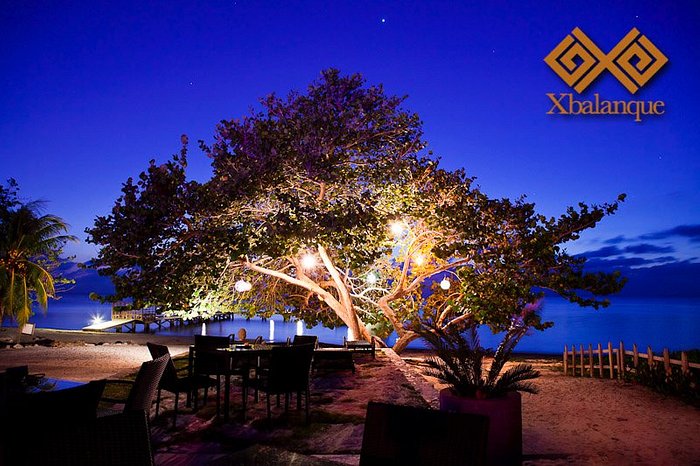The serene image captures a picturesque outdoor setting just after sunset, evoking the feel of a postcard. The backdrop of the scene features a deep, dark blue sky peppered with a few distant clouds, and a singular star or possibly a planet gleaming in the center. Dominating the foreground is a magnificent, large tree with a vast canopy, its branches adorned with glowing lights that create an enchanting atmosphere. Beneath this tree, arranged on the sandy ground, are several tables and chairs, suggesting a cozy dining area. Surrounding these tables is a wooden fence that demarcates the space, adding a rustic charm.

To the right, a small gravel path enclosed by a fence stretches towards the water's edge. The crystal-clear body of water reflects the twilight sky, adding to the tranquil ambiance. Scattered around this idyllic scene are various plants, including a notable small palm in a planter and other tropical foliage, contributing to the resort-like feel of the location. A pier juts out into the water to the left, partially obscured by the tree, while further left, additional palm trees sway gently.

In the top right corner of the image is a logo featuring two gold squares framing the text "XBALANQUE" in yellow, indicating the probable location or branding of the resort area. Overall, the image encapsulates a peaceful, tropical setting perfect for a relaxed dinner by the water under the softly lit canopy of a grand tree.